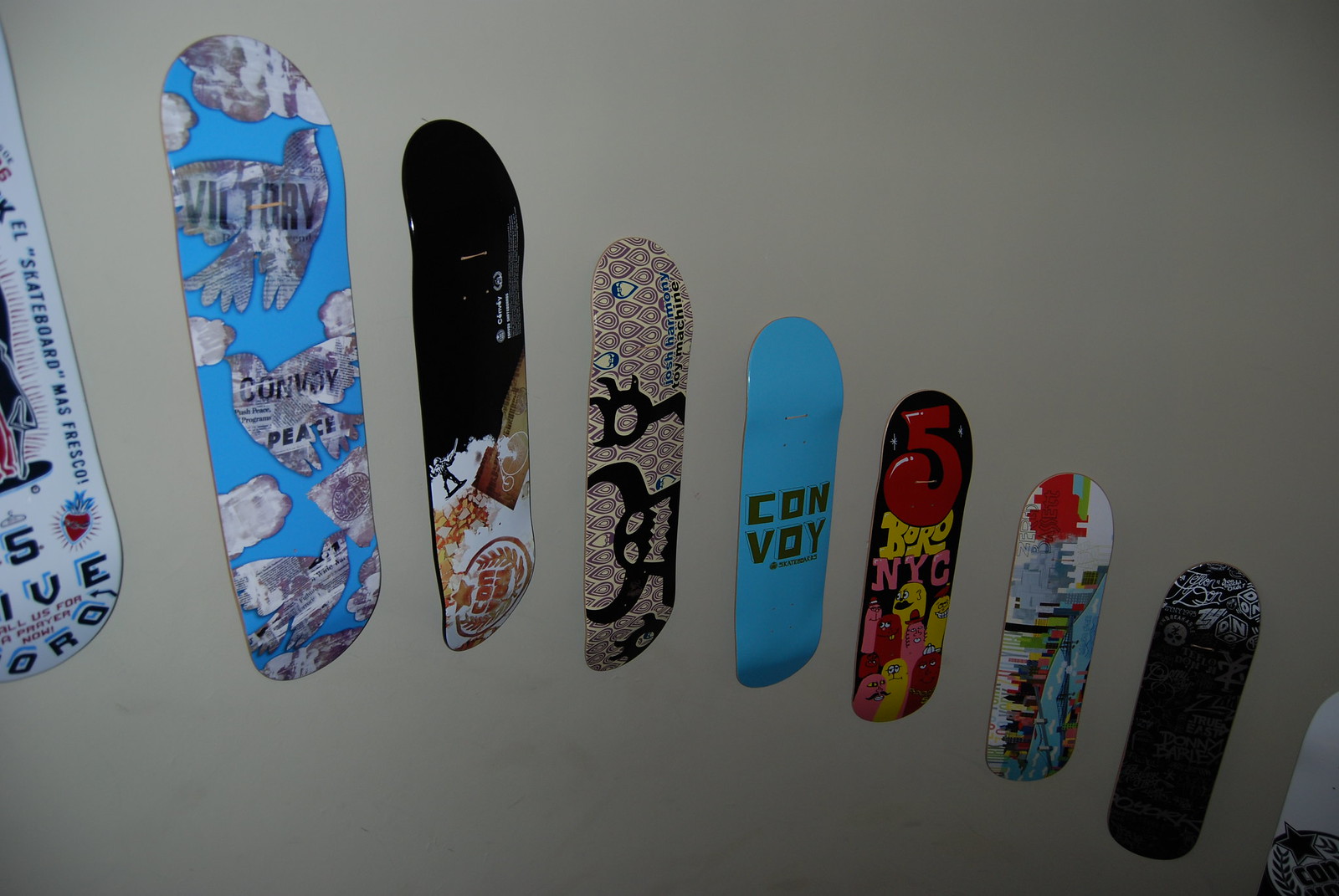This image captures a collection of intricately designed skateboards, sans wheels, arranged in a descending order along the cream-colored wall of what appears to be a staircase. The boards, each unique in design, showcase a diverse array of styles and colors. From left to right, the first, partially out of frame, is a white board with red and dark blue writing, featuring the phrase "El Skateboard Mos Fresco." Following this is a light blue skateboard adorned with silhouettes of birds, their bodies overlaid with newsprint patterns. The next board presents a stark contrast with a black top half and a white lower half, embellished with yellow, gold, orange, and brown designs, including a leaf motif within a circular star emblem.

A multicolored skateboard follows, set against a dark cream background with maroon teardrop shapes and a Viking skeleton figure making an "OK" sign. The subsequent board is sky blue, branded with the word "Convoy" in black letters. Moving along, a striking black skateboard features a large, groovy-font number "5" at the top, followed by the letters "B.O.R.D" in yellow, "NYC" in pink, and a variety of hot-dog-shaped figures in pink, yellow, and red, some sporting hats and mustaches.

The penultimate skateboard boasts a detailed cityscape in shades of blue, red, white, green, and black, depicting bridges and tall buildings intersected by a waterway. The final skateboard in the series is predominantly black, topped with white script and adorned with illustrations of children's building blocks in white. The intricate variety in designs and colors on these boards creates a visually striking display descending along the staircase.